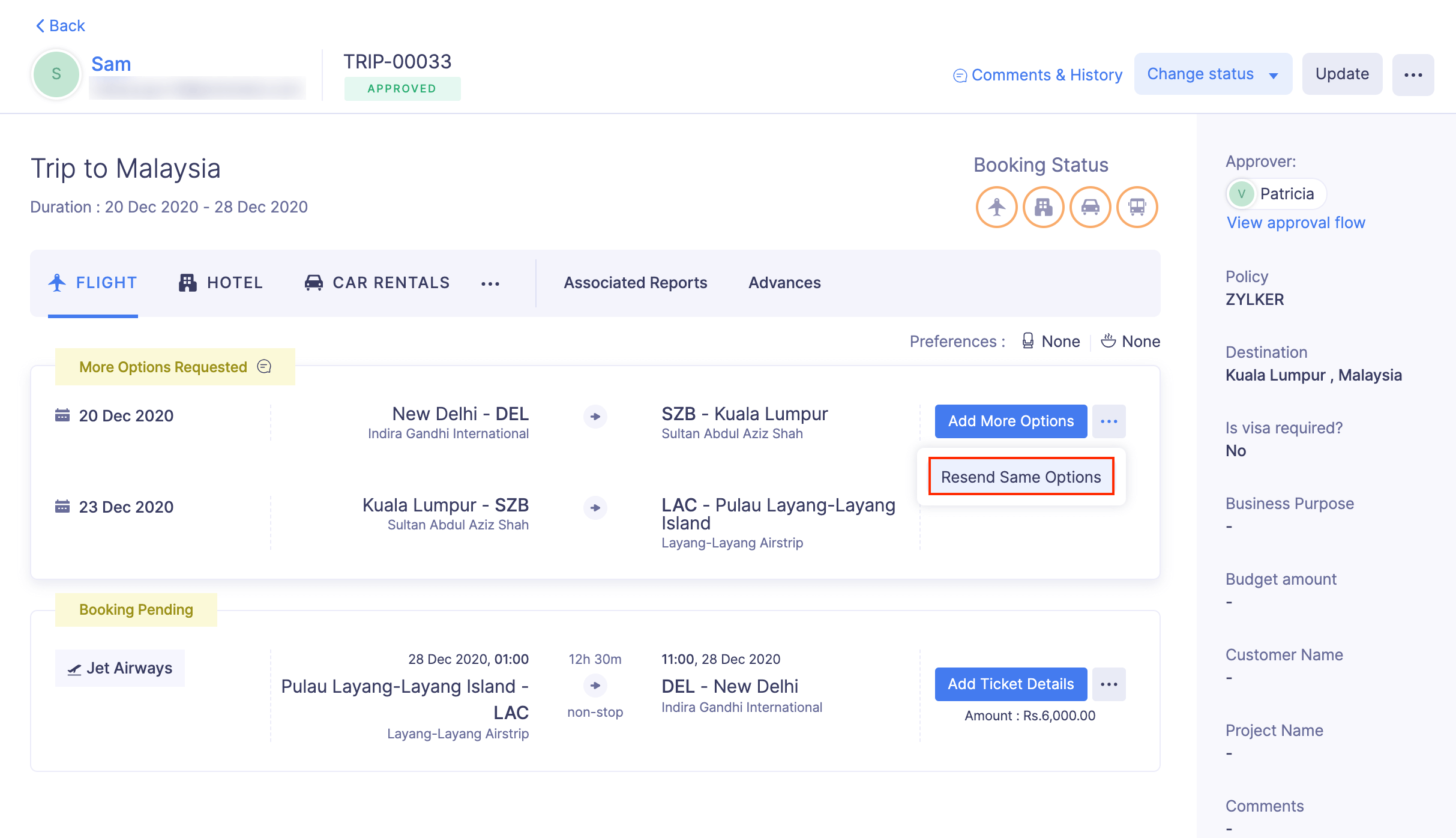Screenshot of Business Trip Information on a Laptop

In the upper-left corner of the screenshot, there is a user profile labeled "Sam." The profile picture is a simple circle with an "S" in the middle, colored light green. The software displayed appears to be a business travel management tool, indicating in the top section that Sam’s trip has been approved by Patricia. 

The trip details for Sam's journey to Malaysia show he is scheduled to depart on December 20th from New Delhi and return on December 28th. The outbound flight is from New Delhi to Kuala Lumpur. Although the specific airline is not listed, comprehensive ticket details are provided, including the departure and arrival airports and the exact times of the flights. 

The visual layout, combined with approval and administrative details, suggests a professional software application specifically designed for managing business travel arrangements.